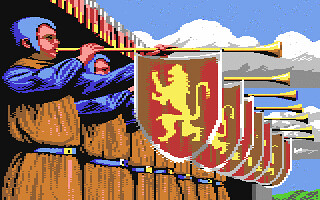This highly pixelated animated image appears to be from an old video game. It depicts a row of seven or eight figures, each adorned in friar-like robes with blue belts, long blue sleeves, and blue caps. Each figure holds a lengthy yellow horn featuring a crest outlined in white. The crest is distinguished by brown and red stripes with a yellow lion emblazoned at the center. The background showcases a blue sky adorned with white clouds, which are shaded light gray in the middle and darker gray at the bottom, adding depth and atmosphere to the scene.